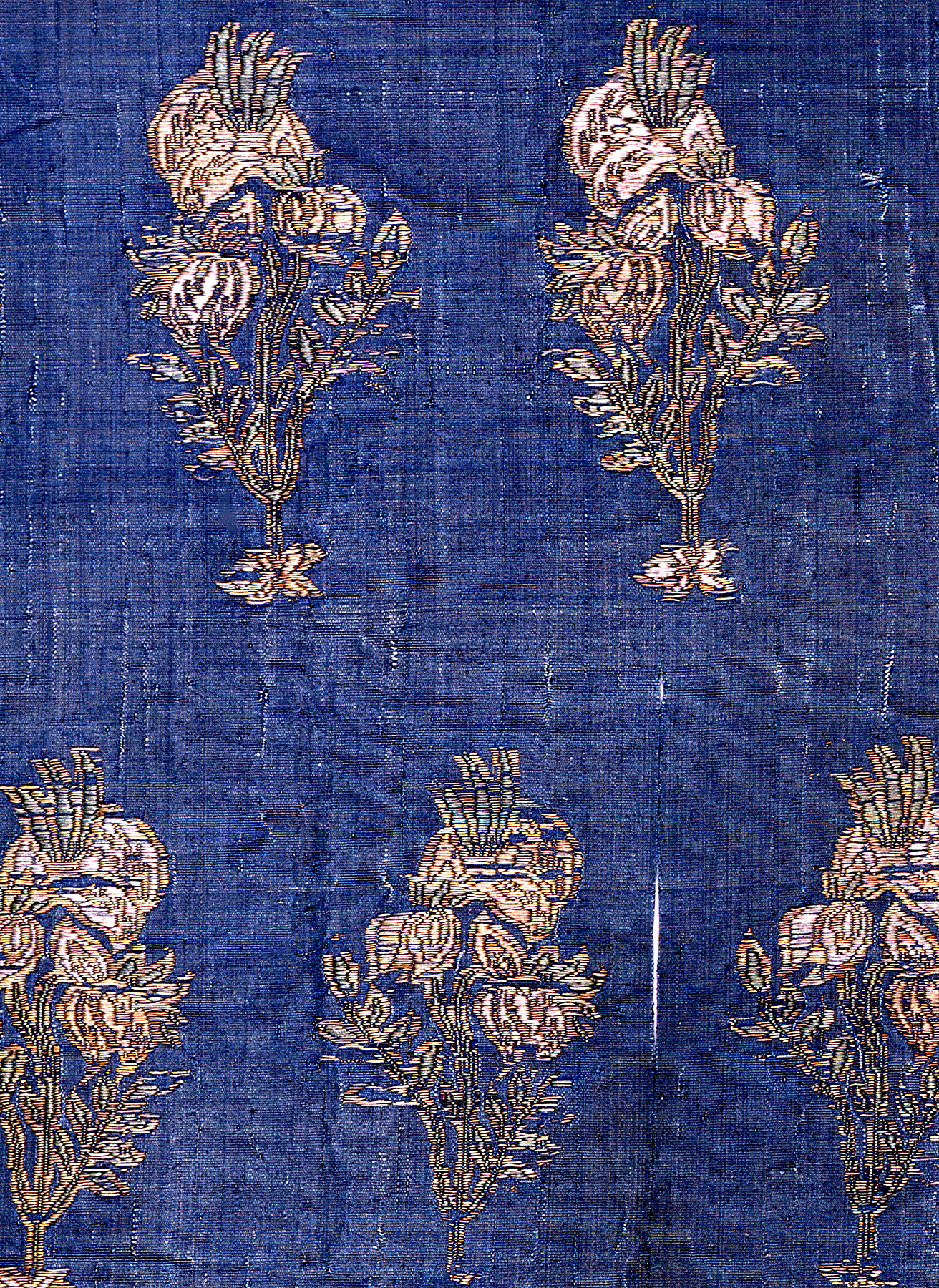The image displays a blue denim-like piece of cloth with a mixture of dark and light blue streaks. The fabric is loosely woven, allowing some white light to shine through in various places. A visible seam runs along the bottom right corner, with light filtering through. The cloth is adorned with intricate embroidered designs predominantly featuring flowers. There are two floral designs at the top and three more at the bottom, all staggered in rows. The embroidery threads are colored in light teal, light pink, light cream, light gray, and black. The flowers exhibit detailed elements such as stems, upward-folding petals, and three hair-like extensions at the top. The bottom part of each flower resembles a stylized, butterfly-star shaped platform. Additionally, the fabric shows signs of wear, with noticeable rips scattered across its surface. Despite some abstract interpretations, the overall ornate design and the combination of textures and colors make it a detailed and visually interesting piece.